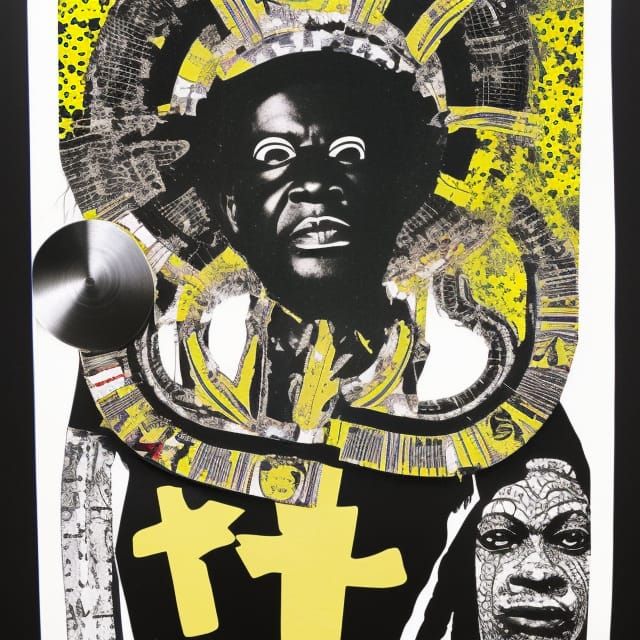The image depicts an artistic rendition of what appears to be an African tribesperson or chief, central to the composition, with a complex, symbolic aesthetic. His face is primarily jet black and partially photographic, overlaid with stylized, cartoon-like eyes rendered in stark black and white. His expression is striking and intense, with wide-open eyes, flared nostrils, and an open mouth that reveals his teeth. Adorning his head and neck is an elaborate headdress or crown that incorporates gray, yellow, and black elements, lending a regal yet abstract quality to his appearance.

His attire mainly features black and yellow, most notably with two prominent yellow crosses on his chest, reminiscent of some cultural or possibly religious significance. A round silver emblem is displayed in the center of his garment. The background of the image maintains a subdued palette of black, yellow, white, and limited red and gray hues that enhance the focus on his form.

To the bottom right of the image lies another face, seemingly a sculptural element or a figure with painted features, which adds another layer of depth to the composition. This face, exhibiting war paint-like markings with dreadlocks, appears lifeless and monochromatic, contrasting with the intense vibrancy of the central figure. Together, the elements meld into a richly detailed and textured piece of art that echoes traditional African motifs while introducing a contemporary, almost surreal twist.